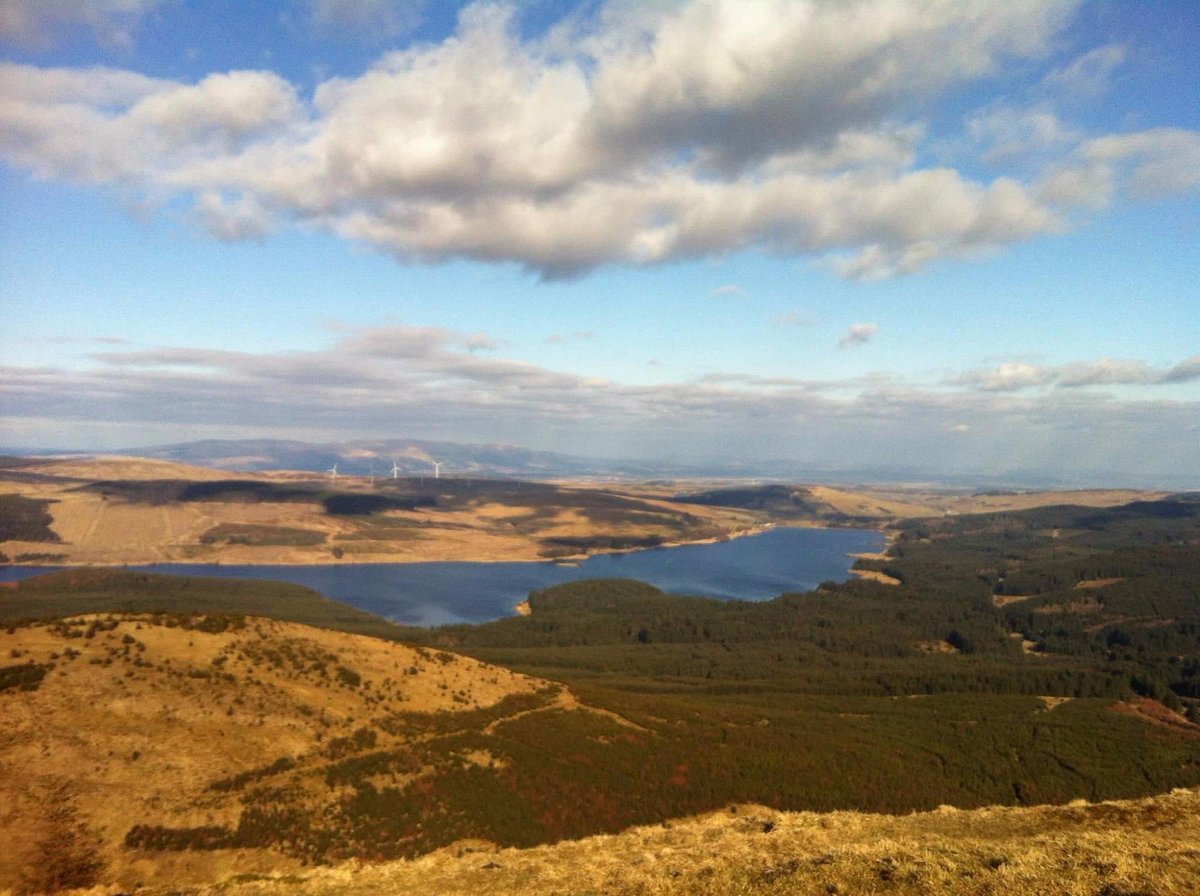This is a beautiful, realistic aerial landscape photograph, possibly of Tasmania or a similar terrain. The image captures a peaceful scene with a clear blue sky, adorned by a few puffy white clouds casting light shadows. The landscape is composed of gently rolling hills, predominantly covered in brown, dried grasses interspersed with patches of dark and light green vegetation, which may be trees or hedges. Central to the image is a tranquil blue river that winds through the hills, creating a striking contrast against the earthy tones. Far off in the distance, three modern white wind turbines rise subtly against the horizon, barely noticeable. There are no signs of human presence or structures aside from the turbines, enhancing the natural and serene quality of the scenery. The overall style is reminiscent of classic landscape photography, with the elements harmoniously balanced, emphasizing the raw beauty of nature.